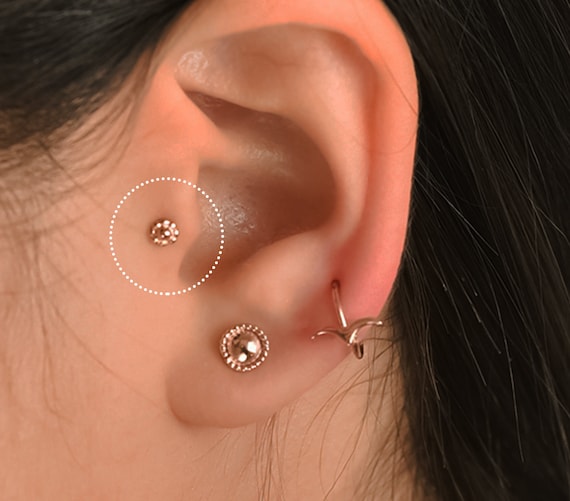The close-up photo captures the left ear of a dark brown, almost black-haired woman with peach-colored skin, who is facing the bottom left of the frame. Her long black hair, swept behind her ear, reveals three distinctive gold earrings. The first is a semi-ring on her earlobe with a design resembling a bird with wings. Above it, another earring in the forward part of the lobe is a circular gold piece with a rim or small studs. Further up in the cartilage, on the outer flap of her ear canal, is a small gold flower septum piercing. This piercing is encircled by a dotted white ring, highlighting its unique placement and intricate detail.